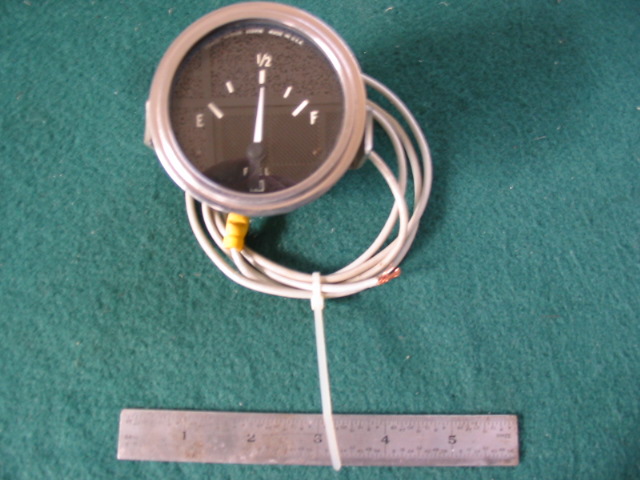The image depicts a fuel gauge with various intricate details. The gauge features a semi-circular dial marked with indicators for "E" (Empty), "F" (Full), and a midpoint labeled "1/2". A white needle points precisely to the half-full mark. Surrounding the dial is a silver bezel. Beneath the gauge, a white wire coils in a circular pattern, leading to a frayed copper end on the bottom right, secured by a zip tie. Additionally, the gauge is partially obscured by a piece of teal cloth in the background. A sequence of numbers, "1, 2, 3, 4, 5," is visible on the gauge's face. A small yellow wrap is noticeable beneath the silver bezel. At the bottom of the image, there is a roller.